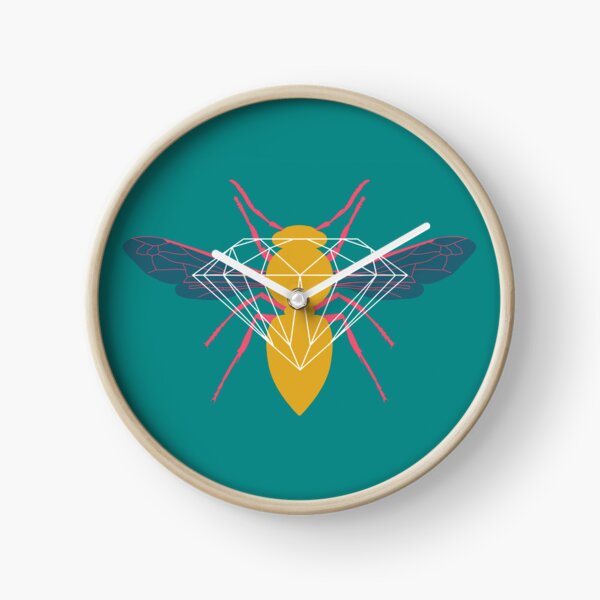The image features a circular wall clock mounted on a white background, with a soft drop shadow towards the bottom right. The clock boasts a minimalist design with no numbers or ticks, and its hands are white. The frame of the clock appears to be light wood or beige, giving it a natural, warm look. The face of the clock has a modern, teal-colored background. At its center is an illustration of an insect resembling a bee or wasp, characterized by a yellow body, pink antennae and legs, and dark blue wings with pink veins. Superimposed on the insect is a white outline of a diamond, adding a geometric element to the design. The clock hands indicate a time a little after 9:10.